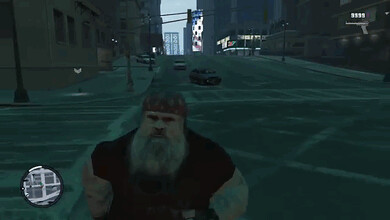This image captures a first-person perspective from a video game, showcasing an urban street scene tinged with a dark gray and blue filter. Dominating the bottom left corner is a man with a gray beard, wearing a hat and a black shirt, standing prominently close to the camera. The scene also includes several cars and clear white lines marking an intersection. A circular minimap is visible, aiding navigation, while the top right corner displays an icon of a gun accompanied by an ammunition count, hinting at the game's action-oriented nature. The overall atmosphere is shadowy and tense, immersing the viewer into the gritty, virtual world.